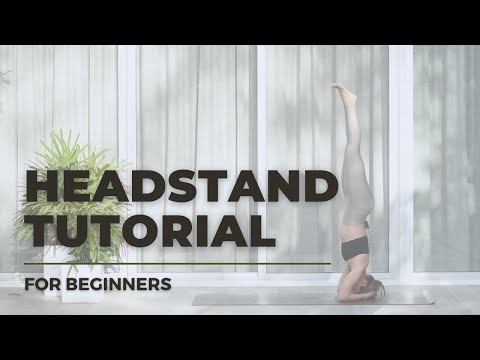The thumbnail for a YouTube video titled "Headstand Tutorial for Beginners" features a detailed image of a woman demonstrating a headstand yoga pose. The text on the thumbnail is bold and prominent: "Headstand Tutorial" in large letters with "For Beginners" in a smaller font beneath it. The woman, positioned towards the right side of the image, is balanced on her head with her forearms on a silver yoga mat, her legs perfectly vertical. She is dressed in a black tank top and white yoga pants, showcasing excellent form and focus. Surrounding her, the background reveals white wood-paneled walls, contributing to a clean and serene atmosphere. On the left side of the photo, a large potted plant with verdant, spiky leaves in a white pot adds a touch of natural greenery. The top and bottom of the image are bordered by thick black bars, creating a framed look. This carefully composed thumbnail aims to attract beginners looking to learn the basics of headstands in yoga.